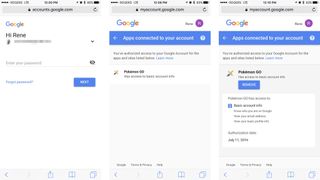**Detailed Caption:**

The image consists of a sequence of small screenshots depicting a login interface, likely belonging to a Google service. Due to the diminutive size of the screenshots, the text is challenging to decipher with precision. However, in the first screenshot, the page appears to display a greeting message, possibly "Hi," followed by a prompt to "Enter your password" with a "Next" button positioned to the right side of the screen. The second screenshot, centrally placed within the image, features a blue banner at the top, which could be indicative of a notification or informational message. Below this banner, there seems to be a descriptive text section, although the exact content is unclear. The third screenshot on the right mirrors the format of the first, showing another text box containing more information. The overall layout and design elements are characteristic of a standardized Google login or account-related page.